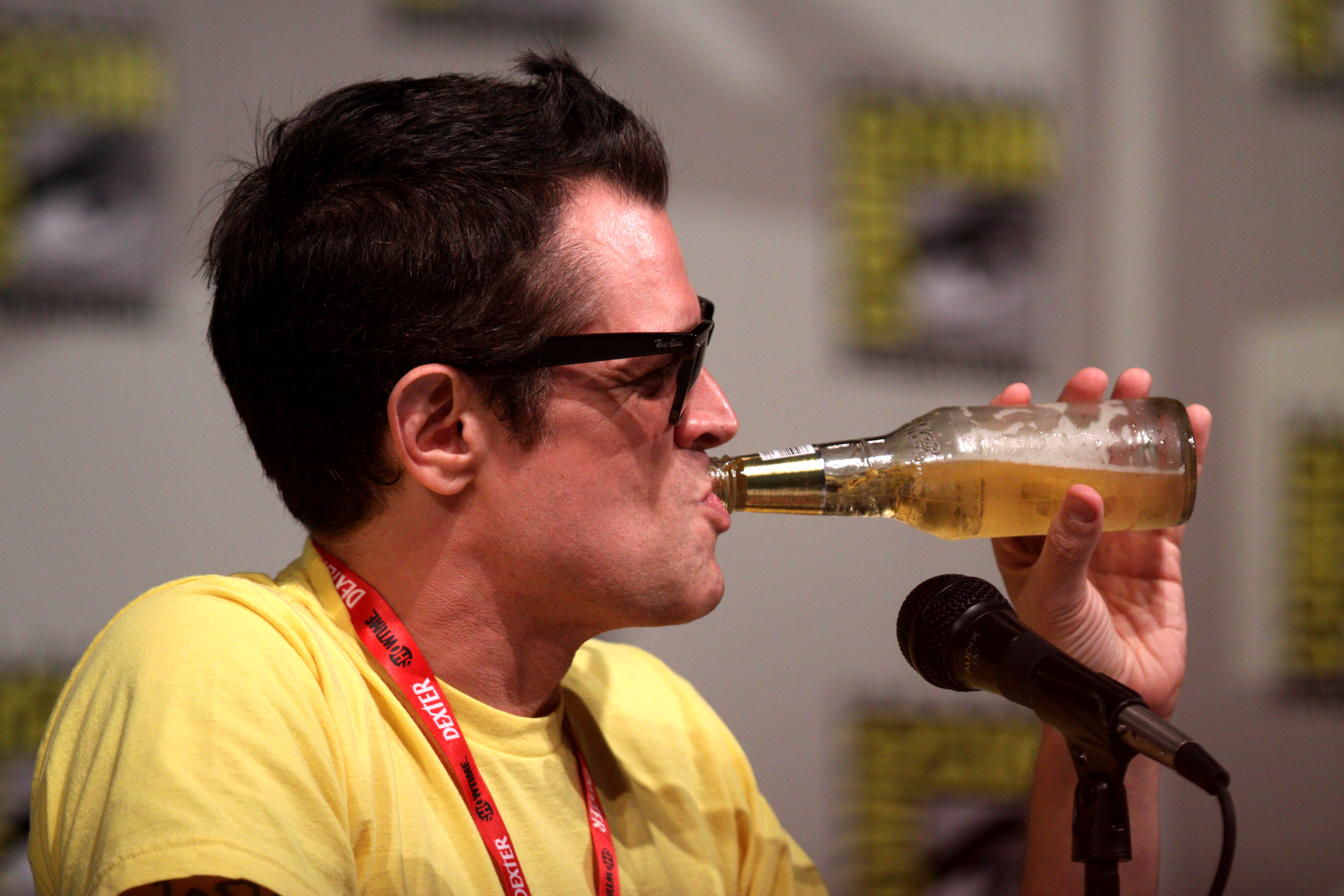This photograph captures Johnny Knoxville seated at a podium during a Comic-Con panel, recognizable by the blurred white Comic-Con logo in the background. He is seen in profile, casually sipping a beer from a gold, yellowish bottle with white suds, indicative of a typical beer. Johnny, with his short black hair styled up in the front, sports black Ray-Ban glasses and has distinctive sideburns. He is wearing a yellow t-shirt and a red lanyard around his neck that reads “Dexter Showtime.” The black and silver microphone in front of him suggests he's engaged in a panel discussion. He appears to be smiling slightly, with squinted eyes, adding a relaxed and cheerful vibe to the scene.